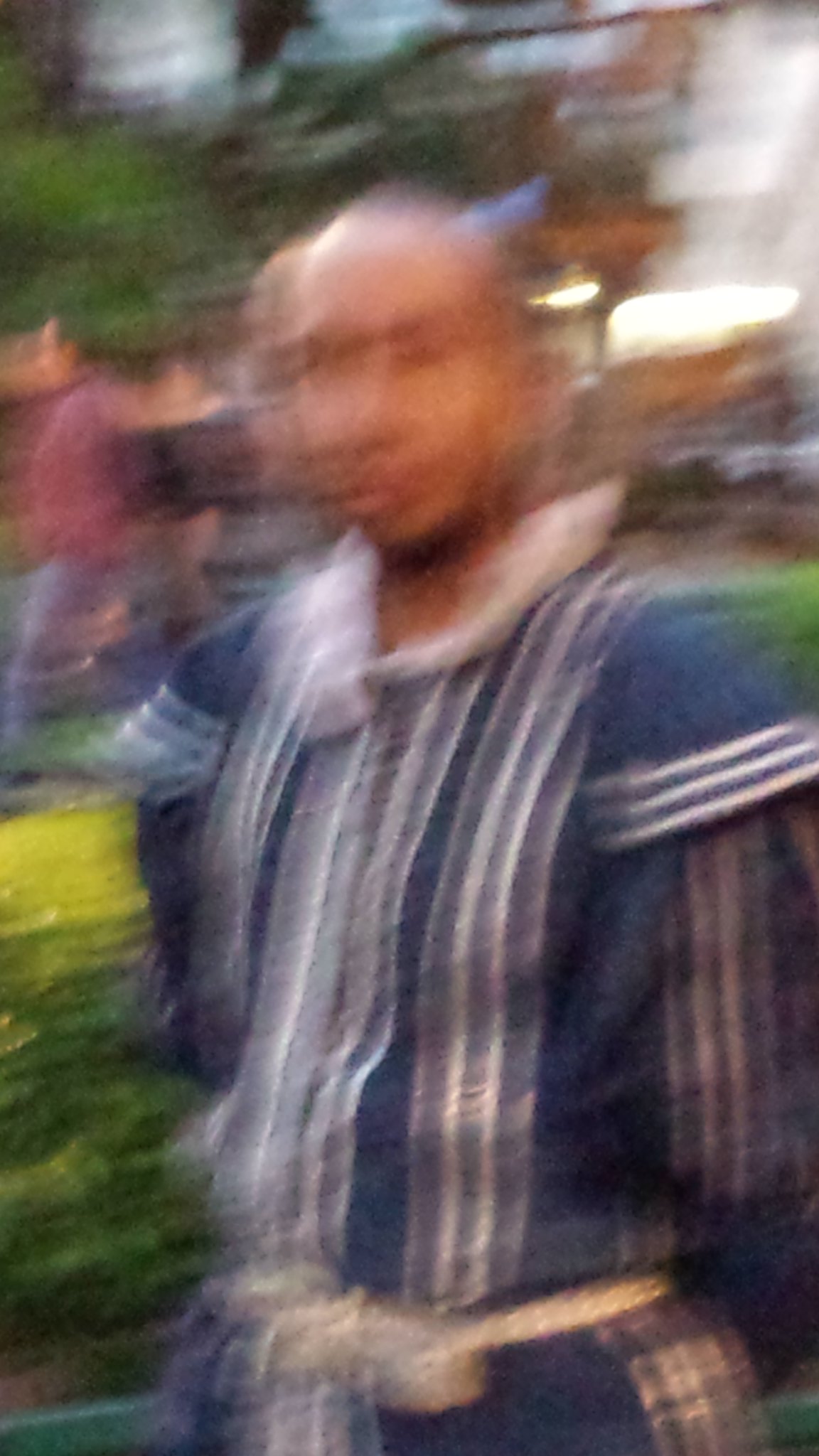This is an exceptionally blurry photograph of a bald man with light brown skin, standing from just below the waist up and facing the camera. He is dressed in a dark blue, robe-like medieval-style outfit adorned with vertical white stripes and frilly, ruffled trimmings. A white sash or rope is tied around his waist. The image captures the man with his head slightly blurred due to movement, making his facial features indistinct. He appears to have his hands behind his back. In the somewhat out-of-focus background, there are visible elements including hedges, possibly buildings or trees, and two people walking, all bathed in a light that suggests it might be early evening. The main colors in the background are a mix of green, red, and white.